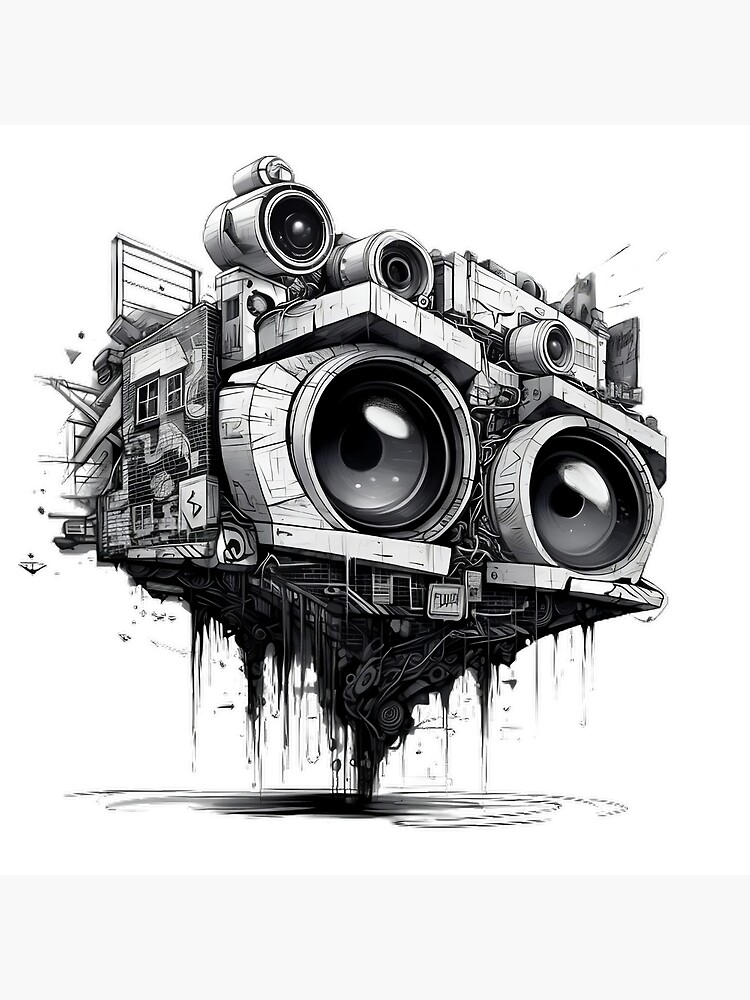This intricate black and white line illustration depicts a futuristic sci-fi robotic station that closely resembles a mechanical face. The focal point is a pair of large, eye-like lenses, akin to binoculars, facing outward that immediately capture attention. These 'eyes' are framed by curved concrete slabs reminiscent of eyelids, further enhancing the facial appearance. The structure is supported by a complex array of machinery and electronics that converge into an upside-down funnel shape at the base, which appears to hover above debris and hanging cables. Alongside this mechanical visage, there are elements resembling windows and walls, suggesting an interior space, while additional building and mechanical components, including what look like engines and rocket propulsion devices, extend above it. The entire composition, full of steampunk elements and drawn in a highly detailed, comic-like style, evokes a scene from a sci-fi universe, with hints of organic matter hanging from its base, giving the impression of age and decay.